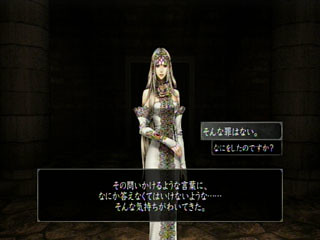This image is a screenshot from a video game featuring a central female character set against a dark background. The character is depicted wearing an elegant, off-the-shoulder dress with long sleeves. She has long blonde hair cascading down her back, and around her neck, she wears either a piece of intricate jewelry or a decorative element that's part of the dress. Upon her head, she adorns a jeweled crown or headpiece that adds to her regal appearance. She is standing still, facing slightly to the left. Additionally, there are various boxes next to her filled with text in a non-English language, contributing to the game's immersive and possibly fantastical setting.